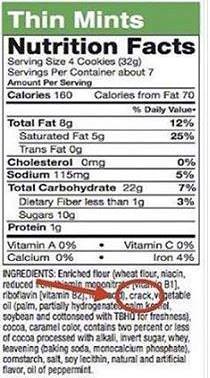The image displays the nutritional facts label of a Thin Mints package. The label is set against a white background with black lettering and borders, featuring a thin green border at the top with "Thin Mints" written in white print. Underneath, "Nutrition Facts" is prominently displayed in large black letters. The label details the serving size as four cookies (32 grams) with approximately seven servings per container. Each serving provides 160 calories (with 70 calories from fat), and includes: Total Fat 8g (12% DV), Saturated Fat 5g (25% DV), Trans Fat 0g, Cholesterol 0g, Sodium 115mg (5% DV), Total Carbohydrate 22g (7% DV), Dietary Fiber less than 1g (3% DV), Sugars 10g, Protein 1g, Vitamin A 0%, Vitamin C 0%, Calcium 0%, and Iron 4%.

The ingredient list includes enriched flour (with various vitamins such as niacin, riboflavin, and vitamin B1), vegetable oils (soybean and cottonseed), cocoa processed with alkali, caramel color, invert sugar, whey, leavening agents (baking soda and monocalcium phosphate), cornstarch, salt, soy lecithin, natural and artificial flavors, and oil of peppermint. Notably, there is a red circle and red arrow pointing to the word "crack" prominently displayed within the ingredients section, which obscures some other ingredient details.